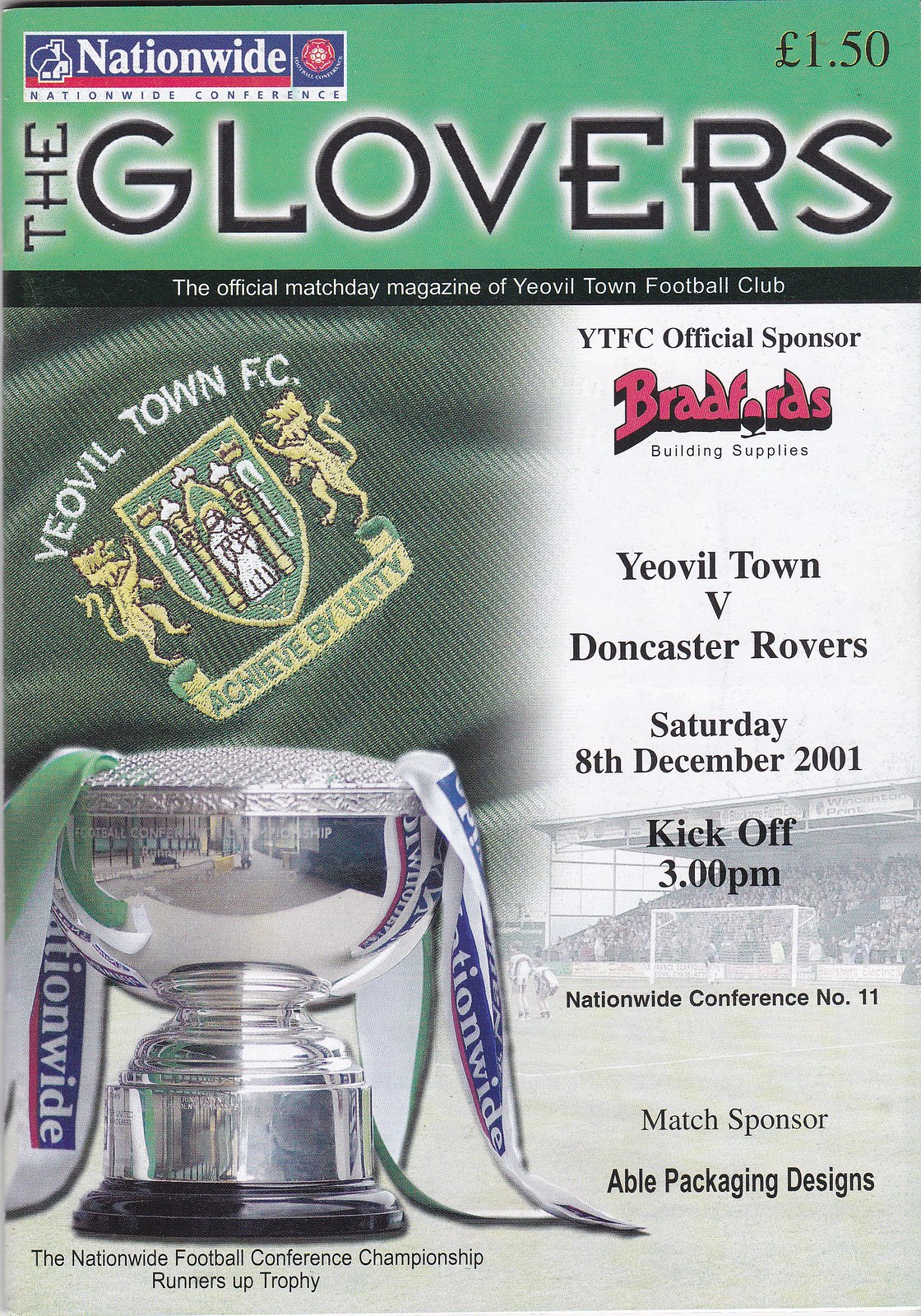This image is the cover of "The Glovers," the official match day magazine of Yeovil Town Football Club, priced at £1.50. The background is green at the top, with the title "The Glovers" prominently displayed in black letters. Below the title, the text indicates that it is the official match day magazine for Yeovil Town FC. The central feature of the cover is a close-up of the Yeovil Town Football Club crest, embodying the motto "Achieved by Unity," printed on what appears to be uniform material. Below the crest, there is a high-resolution image of the Nationwide Football Conference Championship Runners-Up Trophy prominently positioned in the bottom left corner.

On the right-hand side of the cover, the essential match details are outlined: "Yeovil Town v. Doncaster Rovers, Saturday, 8th December 2001, Kickoff 3 p.m., Nationwide Conference No. 11." Also noted is the match sponsor, Able Packaging Designs, and the club's official sponsor. In the background, faintly visible on the lower right side, is an image of bleachers filled with football fans in a stadium, set behind a football field with goalposts.